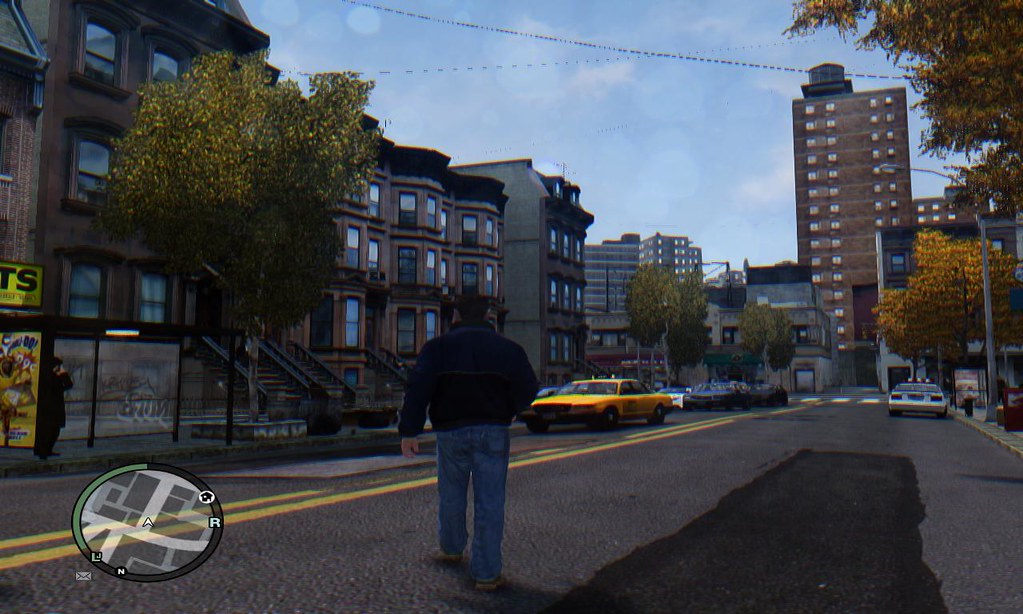A screenshot from a video game depicts a bustling city scene. In the bottom left corner, a circular mini-map illustrates various roads and buildings, with a green segment on its left side and the remainder in black. Dominating the center, the main character is dressed in blue jeans, brown shoes, and a navy coat, seen mid-stride as he crosses a busy street. Opposite him is a stationary yellow taxi cab, flanked by a blue car and a white car. Another white car is visible across the street. The surrounding cityscape features older, multi-storied buildings in dark hues of brown and gray. In the distance, a towering high-rise building, also brown, looms large over the scene. Street details include trees, a bus stop, and assorted urban paraphernalia.